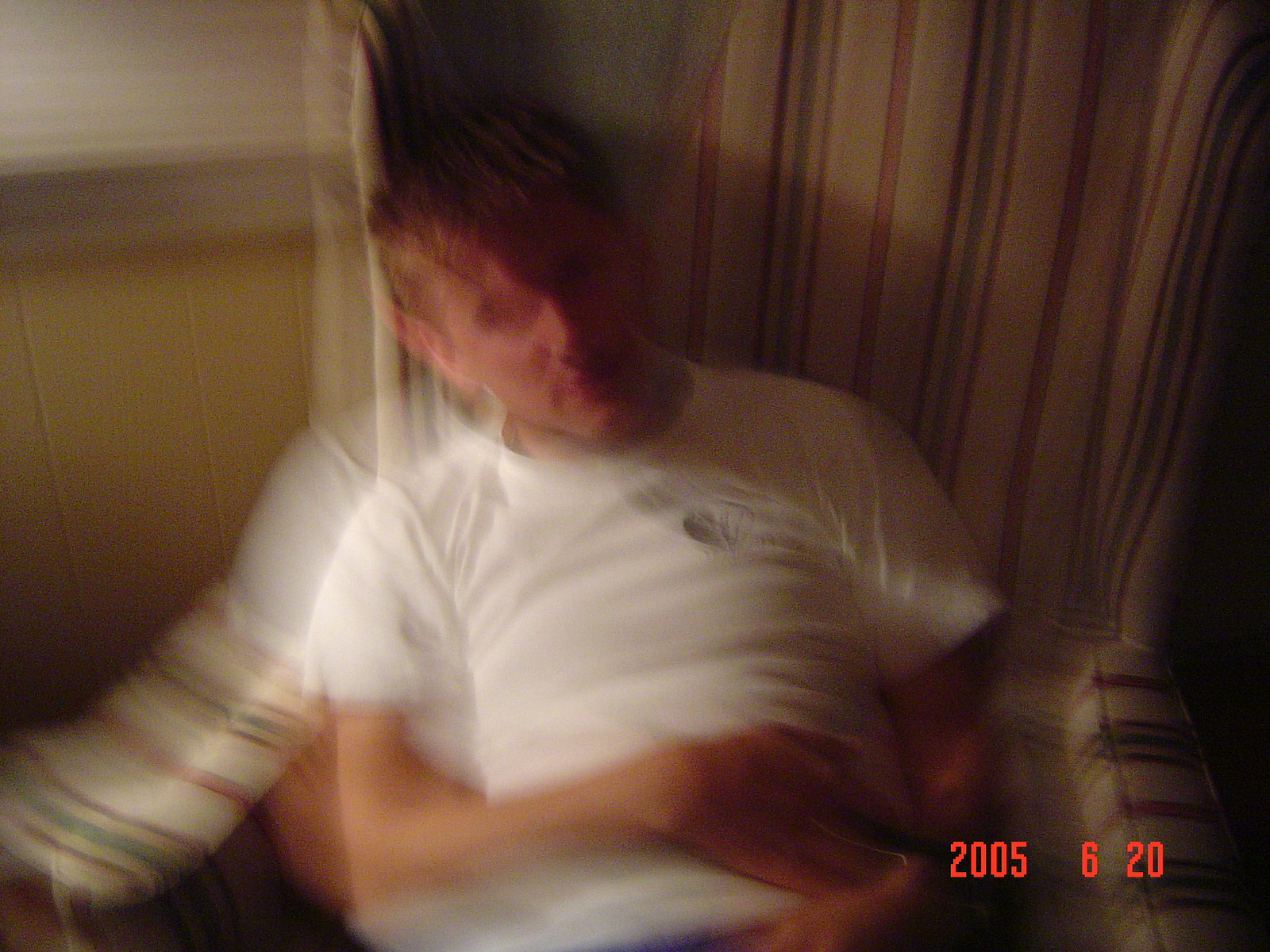The photograph is an indoor, extremely blurry, and out-of-focus color image, appearing to use possibly some time-elapse special effects, giving it a double image effect. Dominating the upper left-hand corner is the edge of a window, accompanied by a vertically hanging curtain that appears to be beige with red and green stripes. In front of this backdrop, a man of Caucasian appearance with short blonde hair is slumped in a large, high-backed, light beige chair adorned with orange, green, red, and blue vertical stripes. His facial features are indistinct, some obscured in shadows, and his head appears bent toward his right, possibly with his eyes closed. He is dressed in a white t-shirt that has a logo on it, with glasses hanging from its collar. His right forearm rests across his stomach, with his left hand not clearly visible, giving the impression he might be holding an indistinguishable object such as a pen, TV remote, or smartphone. A date and time stamp in red is visible in the bottom right-hand corner, reading "2005-6-20."